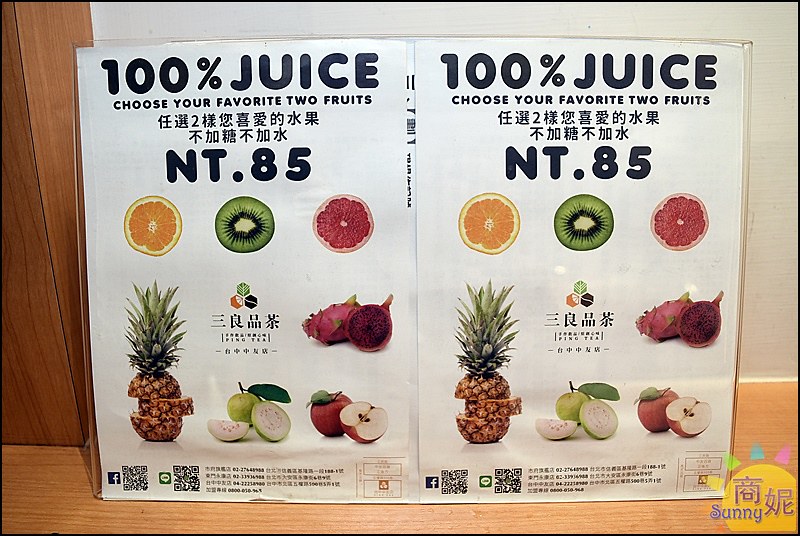The image shows two identical laminated pages featuring a multilingual advertisement, possibly for a magazine, grocery store, or restaurant. The background consists of a white drywall wall, brown wood trim on the left, and a lighter brown surface that could be a tabletop or floor. Each page has a white background adorned with pictures of various fruits, including an orange, kiwi, grapefruit, pineapple, dragon fruit, apple, and pear. The top of each page prominently displays the text "100% Juice" in bold, with "Choose Your Favorite Two Fruits" in smaller text below. Beneath this is a line of Asian characters, followed by "NT.85" in bold. At the bottom are additional Asian characters and two QR codes, one of which includes the Facebook symbol.